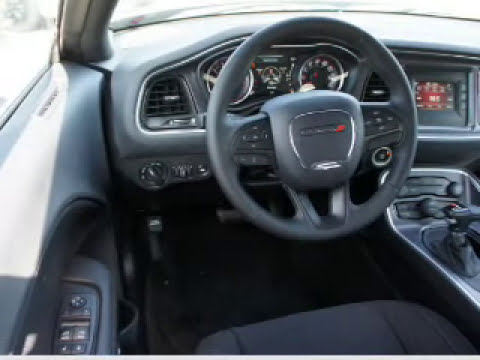The image depicts a close-up view of the driver's side interior of a seemingly high-end vehicle, filling the entire frame. Central to the image is a black steering wheel, situated above a cluster of traditional analog instruments, including a speedometer and various other circular gauges. To the immediate right of the steering wheel, the gear console is visible, alongside the dashboard, which houses controls for the radio and air conditioning. The vehicle appears to be a stick shift, emphasizing its advanced yet traditional setup. Above the gear console, there is a small digital display. The black driver's seat and a bit of the door are partially visible, showcasing the controls for the locks and windows. The high-quality upholstery adds to the impression of a luxurious car. Ambient daylight filters through the barely glimpsed windows, enhancing the richly detailed interior.